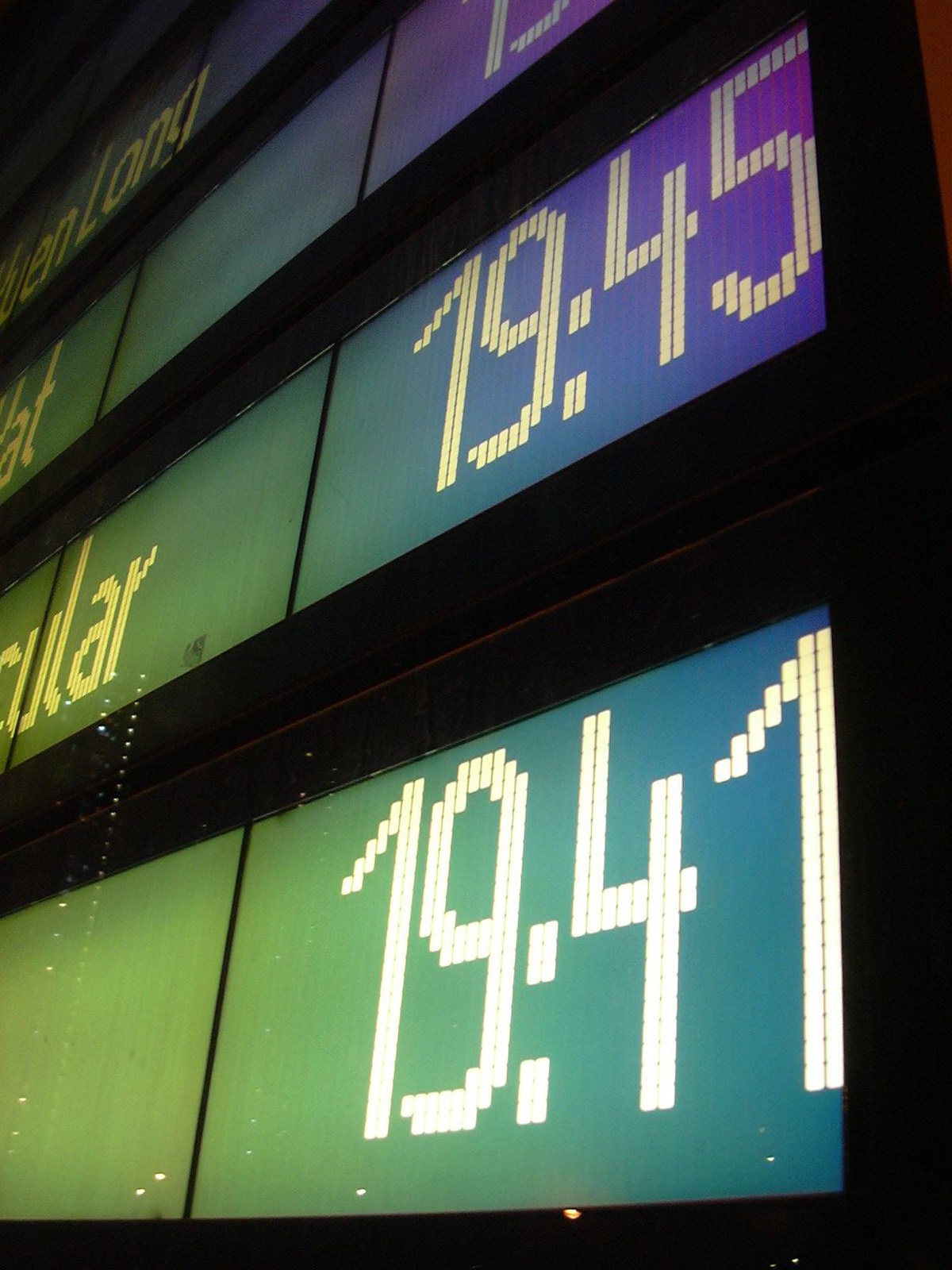This is a photograph taken at an angle, capturing a large, multi-sectioned sign, likely from a train station or airport. The sign is framed with a black border and divided into four horizontal sections, each separated by black lines. The left side of the sections transitions in color from light green to dark green, light blue, dark blue, and finally to purple, from top to bottom. The displayed content, written in white and partially obscured yellow text, includes the fragmented words "long" on the top row, "A-T" on the second row, and "U-L-A-R" on the third row. The number "1945" is visible at the right end of the third row, and "1941" appears at the right end of the bottom row. The background behind these sections is black, and the sign seems to be listing times rather than prices.